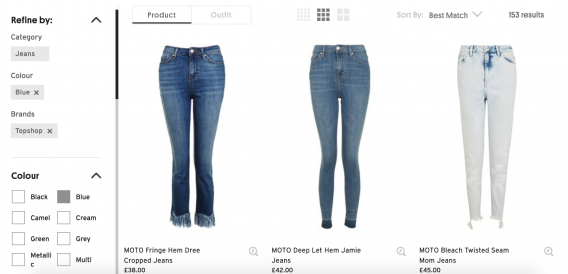Screenshot of an Online Clothing Store:

The screenshot captures an online clothing store interface, set against a clean white background. On the left side, there is a vertical menu titled "Refine By," followed by selectable filters. The first filter is "Category," with "Jeans" entered. Beneath this, the "Color" filter shows "Blue" as the selected option. The "Top Shop" filter is also activated, confirming the products are from that brand. Below a horizontal black separator line is another "Color" filter with clickable options presented as small white boxes. The selected color is "Blue," with other available options including black, camel, cream, green, gray, metallic, and multi.

On the right side, there are search results displaying three pairs of women’s jeans. Each result features an image of the jeans along with a brief description and a price. Additionally, a small magnifying glass icon next to each result allows for more detailed viewing.

1. The first product on the left showcases a pair of women's blue jeans with a fringe at the hem. The description reads "Modo Fringe Hem Dry Cropped Jeans" priced at £38. 
2. The jeans to the right of the first pair are more traditional, lacking fringes, but their specific details are not visible in the screenshot.